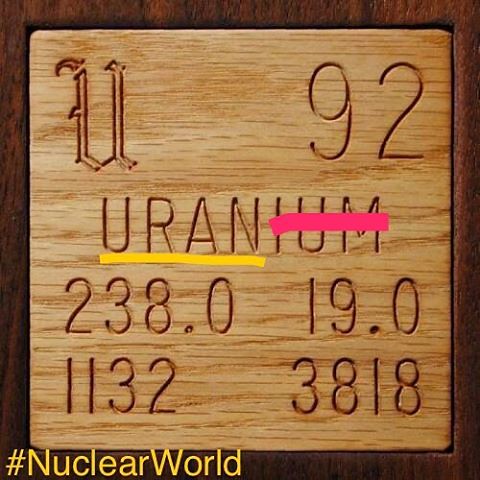The photograph showcases a high-quality, two-toned wooden plaque, with a lighter inner block surrounded by a darker outer frame, likely a permanent fixture in an educational or scientific setting. The plaque prominently features the word "uranium" in the center, with the first four letters "U R A N" underlined in yellow and the last three letters "I U M" strikethrough in thick pink. In the top right corner, the number 92 is etched, while below "uranium," a series of scientific numbers are inscribed: "238.0" on the left, "19.0" on the right, "1132" at the bottom left, and "3818" at the bottom right, possibly referencing scientific data related to uranium. The entire composition is digitally modified with the hashtag "#NuclearWorld" in yellow text, positioned at the bottom left corner of the plaque. The detailed engravings and the rich brown hues of the wood indicate a meticulously crafted piece, potentially located in a science lab or educational institute.